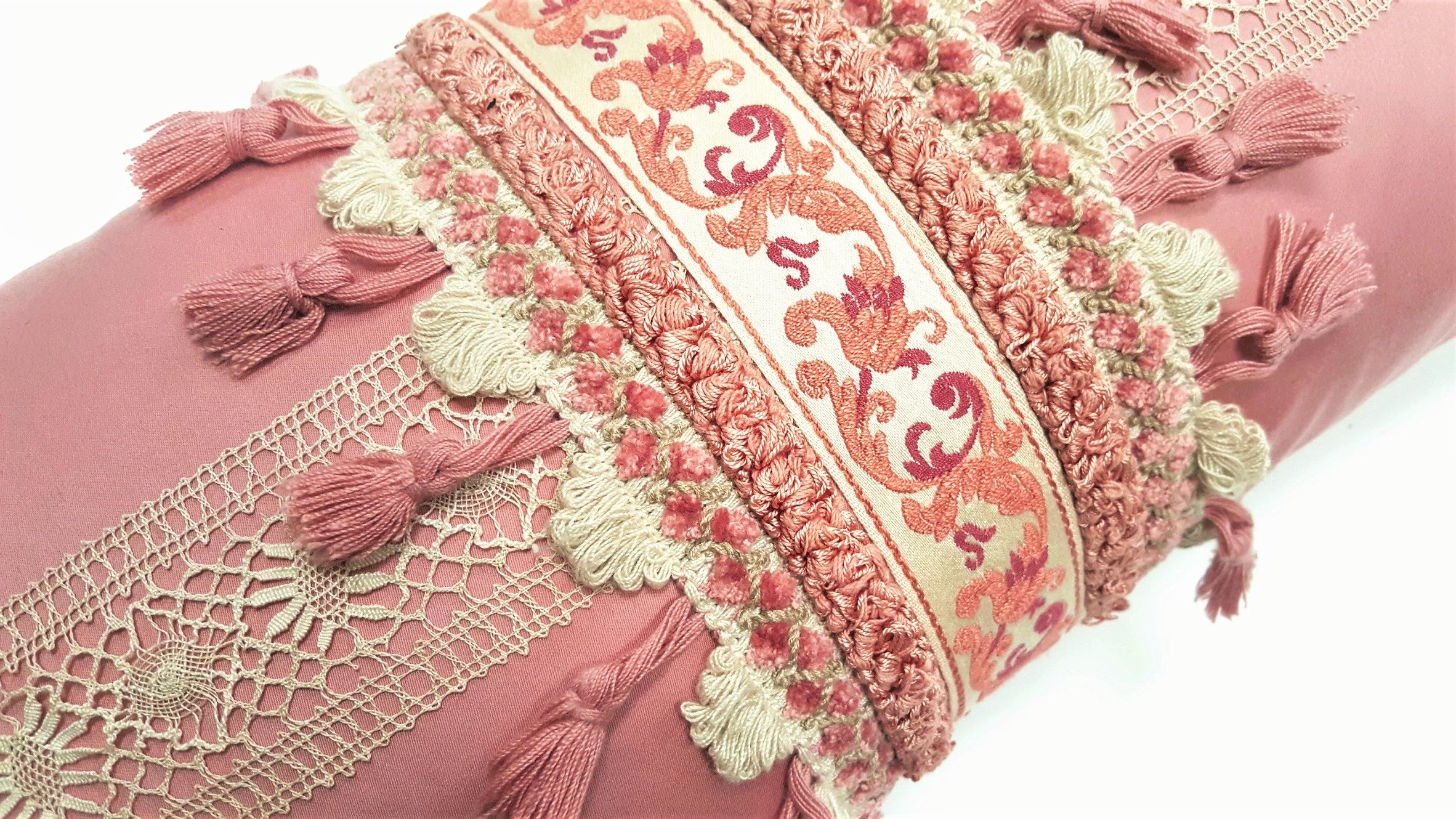The image showcases a tubular pink fabric, possibly a decorative item like a pillow or napkin holder, set against a white or transparent background. The fabric, appearing cylindrical and elaborate, features a central white doily-like runner that spans a third to a fourth of its length. This central piece is bordered by heavily embroidered bands with a pink and peach floral pattern adorned with small pink flowers. Surrounding the embroidered section are loops of pink tassels, four at the top and four at the bottom. The design extends from the lower left to the upper right, framed by additional fluffy, looped pink sections and interspersed beige poofs, creating a complex and ornate textile presentation.